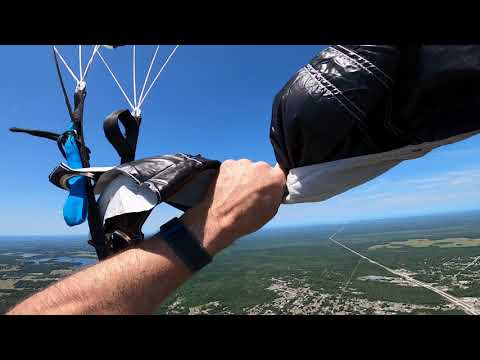The image captures a breathtaking aerial view from the perspective of someone high up in the sky, possibly skydiving, parachuting, or parasailing. The background is dominated by a vibrant, clear blue sky. In the foreground, we see a forearm and hand, likely the left, gripping a black-and-white fabric or pole, which appears to be part of a parachute or parasailing equipment. The person is wearing a black watch on their wrist, and there are additional black straps or handles visible around their hand. Below, the ground is a patchwork of various greens, indicating trees and grass, interspersed with lighter areas that may be water, roads, or rooftops, seen from a great height, reminiscent of the view from an airplane window. The scene highlights the sheer altitude and the freedom of being elevated in the sky, with the vast landscape sprawling beneath.